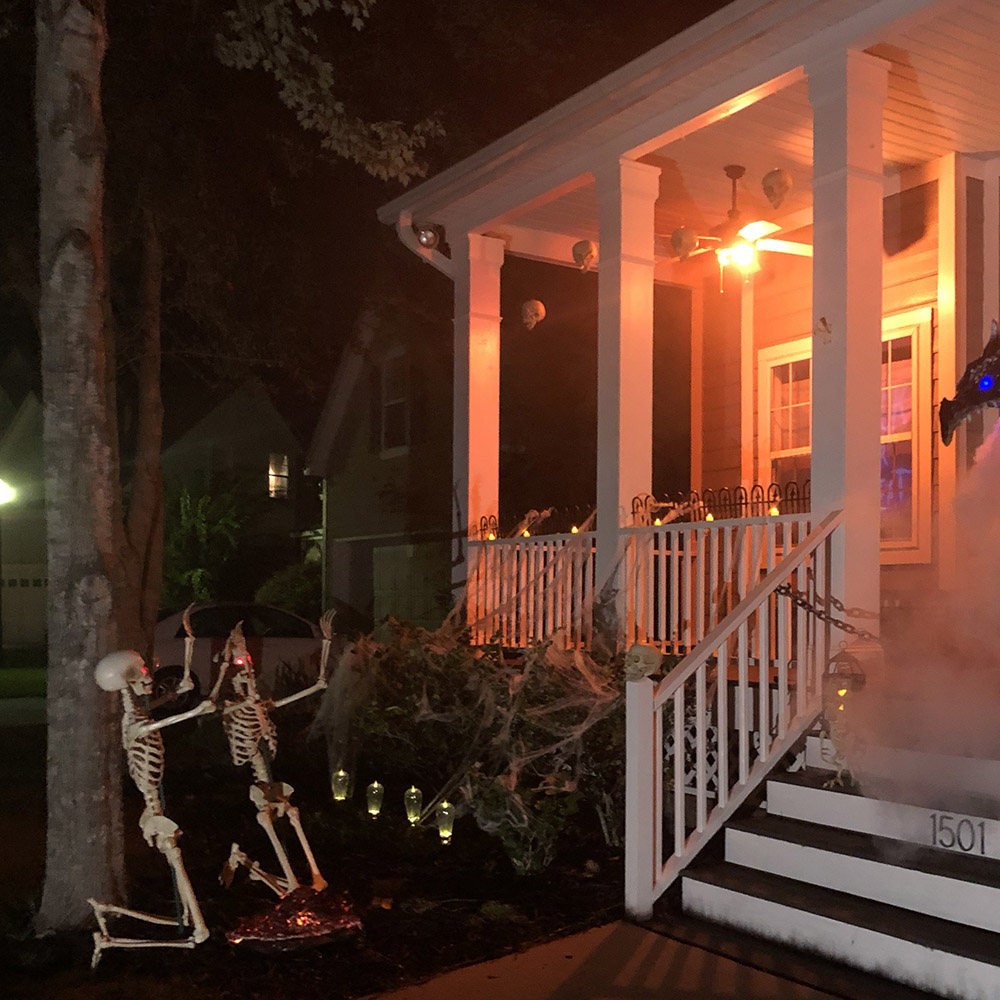This photograph captures an elaborately decorated house porch for Halloween, situated at 1501. The house boasts white-colored walls and matching white stairs leading up to the front door, framed by white railings and pillars. In the night scene, a warm yellow-orange light hangs from the roof, illuminating the porch, while decorative skulls dangle from the ceiling. Dramatically enhancing the spooky ambiance, fake cobwebs drape over the shrubs.

On the left side of the image, two human skeletons with glowing red eyes are kneeling on the ground beneath a tree, seemingly raising their arms in a haunting gesture. An eerie element is the dragon figure on the right side of the porch, which appears to be blowing smoke and has a piercing blue eye.

The house stands out in the neighborhood as the only one adorned for the occasion, with neighboring houses remaining dark and unadorned for the Halloween night.